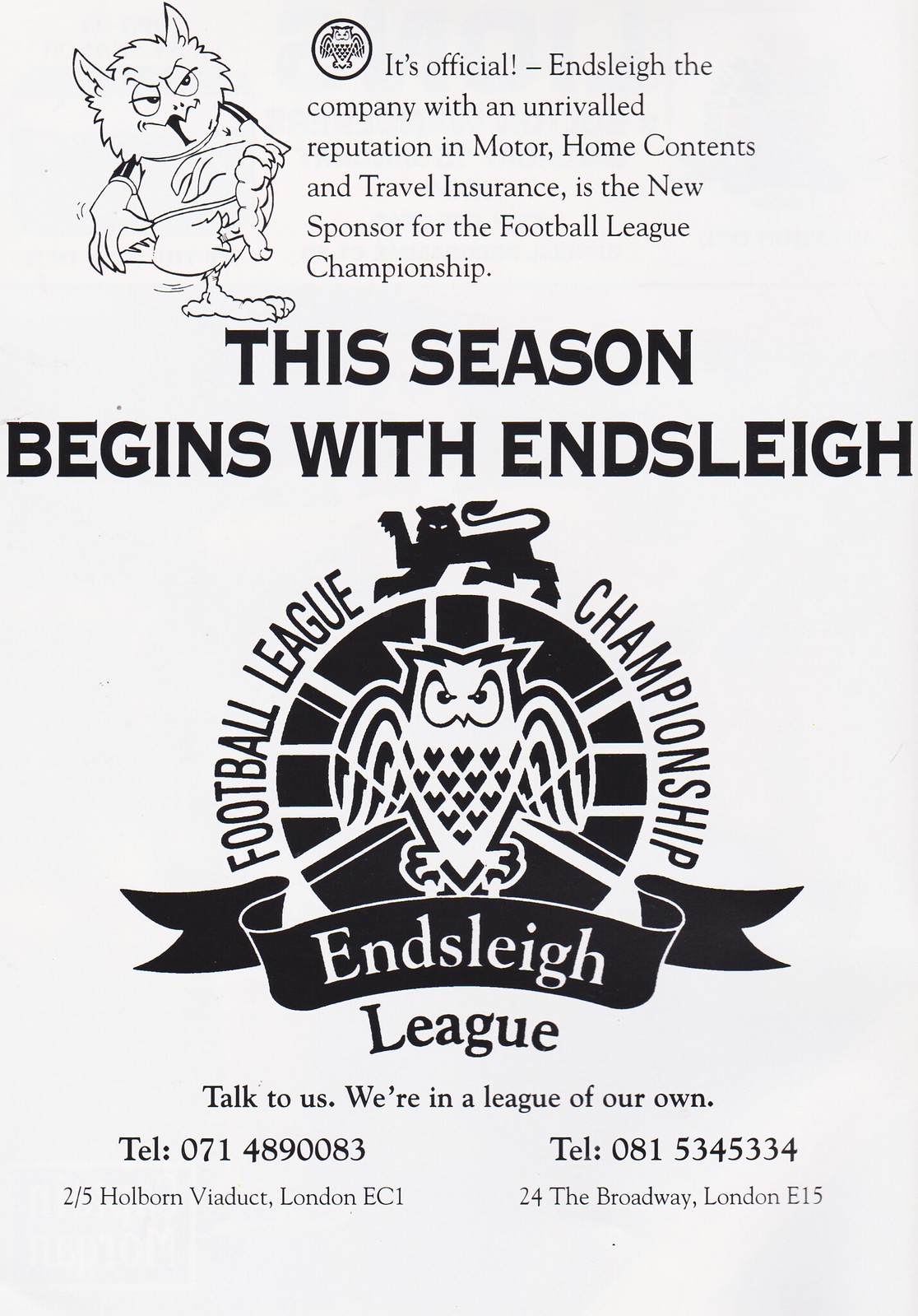The image is a tall, rectangular flyer promoting the Football League Championship, sponsored by Ensley. Set against a slightly light gray background that appears almost tan, the flyer features a black line drawing of an owl in the top left corner. This owl is illustrated wearing a jersey and kicking its foot up, likely serving as a mascot. To the right of the owl, text reads, "It’s official, Ensley, the company with an unrivaled reputation in motor, home, contents, and travel insurance, is the new sponsor for the Football League Championship."

Below this announcement, large all-capital letters in black declare, "This season begins with Ensley." Centered on the flyer is a prominent circular logo featuring an angry owl, with a lion image above it. Encircling the logo in all-capital letters are the words, "Football League Championships." A black ribbon at the bottom of the circle reads "Ensley" in white font.

Towards the bottom of the flyer, additional text states, "Talk to us, we are in a league of our own." A phone number is also included. The overall style of the flyer is a promotional advertisement, primarily utilizing shades of gray and black. Most of the text is positioned towards the top, with the central logo drawing attention in the middle.